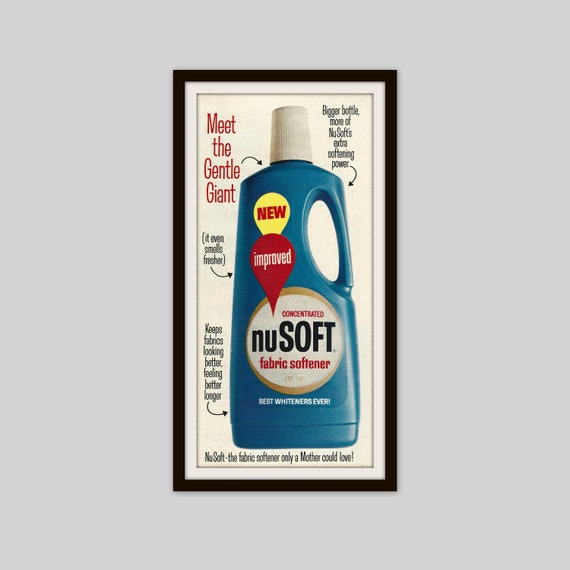This image is a framed photograph of a fabric softener advertisement, framed with a thin black border and hanging on a gray wall, likely as a decorative piece for a laundry room. The centerpiece of the photograph is a blue bottle of "Concentrated New Soft Fabric Softener" with a white cap. The bottle features a yellow sticker labeled "New," and a red sticker on top of it reading "Improved." Surrounding the bottle, various text elements are highlighted with arrows pointing to specific parts of the bottle. 

In the top left corner, red text reads "Meet the Gentle Giant," directing attention towards the bottle. On the right side, another label states "Bigger Bottle, More New Soft's Extra Softening Power," with an arrow pointing to the bottle's handle. To the left side of the bottle, in parentheses, a note says "It Even Smells Fresher," pointing towards the word "Improved" on the bottle. Additionally, on the left side, text claims "Keeps Fabric Looking Better, Feeling Better, Longer," with yet another arrow pointing to "Best Whiteness Ever" on the bottle itself.

At the bottom of the bottle, the main label reads "Concentrated New Soft Fabric Softener," and underneath the bottle, it says, "New Soft, The Fabric Softener Only a Mother Could Love."

The background of the advertisement is cream-colored with a mix of white, black, red, blue, and yellow elements highlighting different aspects of the product’s features and benefits.